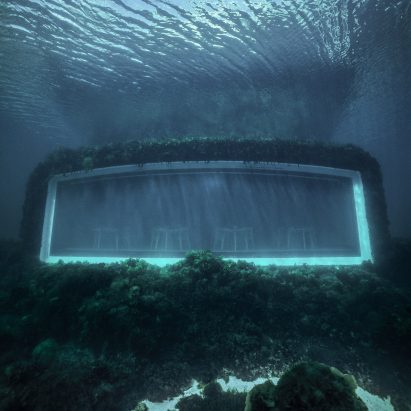This image is an eerie underwater photograph featuring a long-submerged structure that resembles a house with a large viewing window. The house is completely encrusted with barnacles, algae, and other underwater growth. The image is predominantly dark blue, with minimal sunlight penetrating from the surface, creating a dim, mysterious atmosphere. The top part of the photo captures the surface of the water, depicting faint crevices and movement waves. The large window, framed by a white border and covered in moss, dominates the frame. The window is rectangular with a slightly curved top edge, adding to the intrigue. Through the murky glass, four shadowy objects that might be tables or barstools are barely visible. The dark and unclear visibility of the photo leaves much to the imagination, but it evokes a haunting sense of a long-forgotten underwater world.